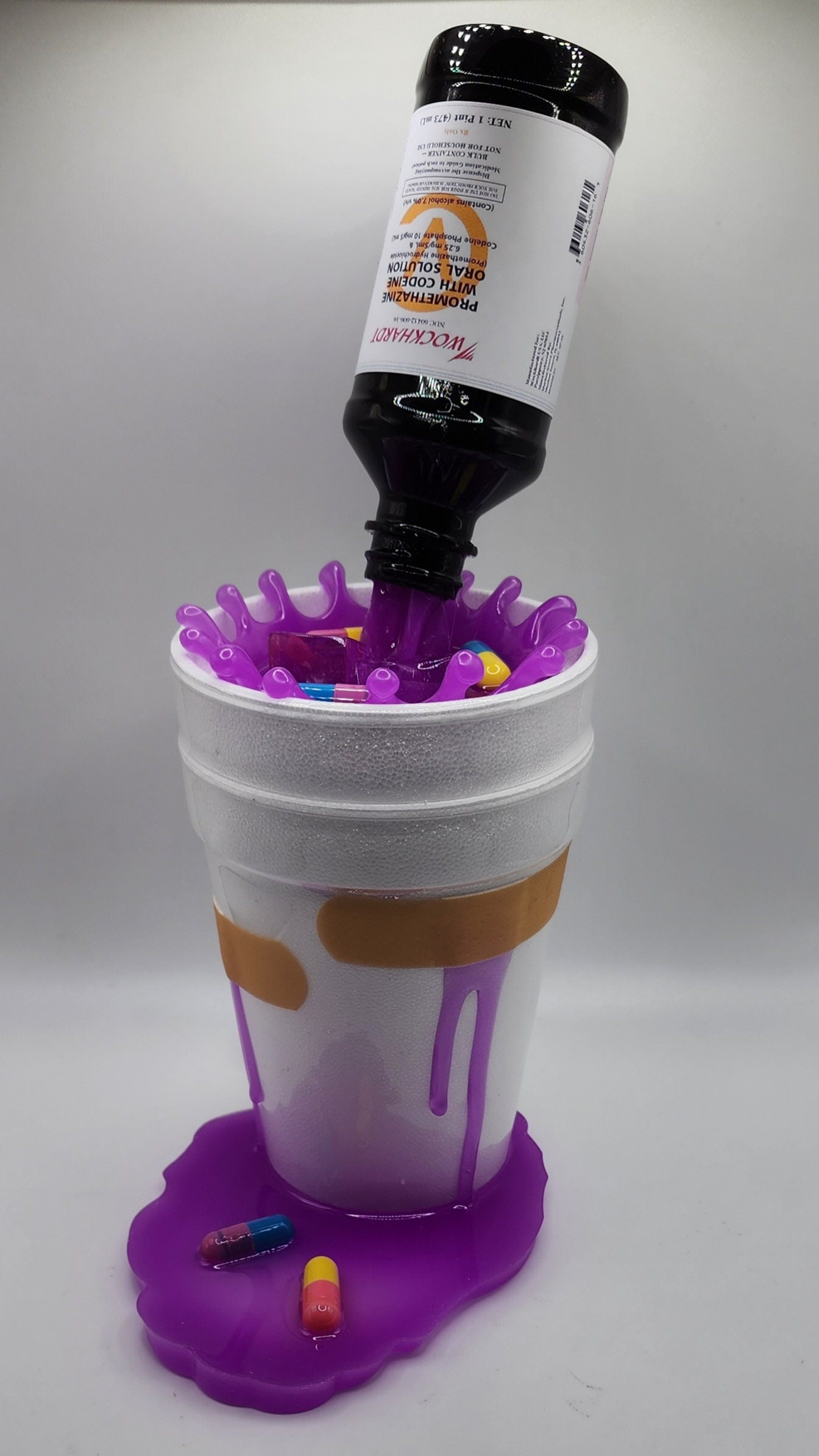The image showcases an intricate sculpture with a medical theme, featuring two styrofoam cups stacked one inside the other. The cups are conjoined and have purple liquid, which is a plastic mold meant to resemble liquid, pouring from an upturned dark-colored cough syrup bottle with an orange symbol on its white label. The liquid cascades into the cups, splashing dramatically out of the top, and dripping down the sides through bandaged holes, creating the illusion of spillage. This faux liquid pools at the base of the cups, forming a thick purple puddle. Immersed within the puddle and within the liquid inside the cups are various colored pills: a yellow and red capsule, a purple and blue capsule, and additional pills that are pink and yellow, and yellow and blue. The sculpture is set against a stark black background with a black surface below and a white wall behind, emphasizing the vibrant colors and intricate details of the piece.